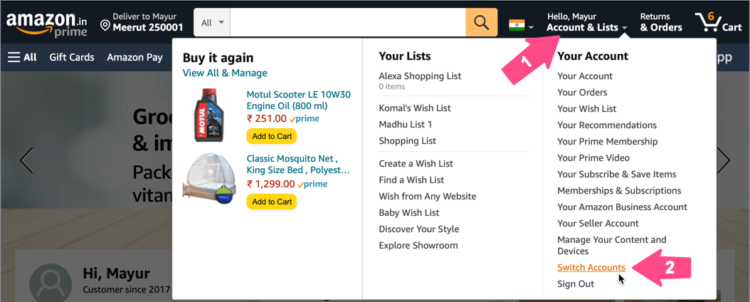Here is a detailed and cleaned-up caption for the screenshot:

---

A screenshot of Amazon's Indian web page, identifiable by the ".in" domain at the top left corner. The page is personalized for a user named Mayur, with the delivery location set to Meerut, PIN: 25001. The top navigation bar includes an Amazon Prime badge beside the greeting "Hello, Mayur" under "Accounts & Lists", which has a drop-down menu opened. A pink arrow labeled with a white "1" points to the "Accounts & Lists" tab.

To the right of the "Accounts & Lists" tab are "Returns & Orders" and a shopping cart icon depicting six items already in the cart. The content of the drop-down window is shown in white and offers various account-related options such as:
- "Buy It Again" section displaying items like LE10W30 engine oil (800 milliliters) priced at ₹251 with Prime shipping and a 'Classic mosquito net for a king-size bed' made of polyester priced at ₹1,299, also with Prime shipping.
- Other account management options, including "Order Lists," "Alexa Shopping List," "Komal's Wish List," "Madhu List One," and more.

There are options to:
- Create and find wish lists.
- Discover style and explore the showroom.
- Manage various account settings such as "Your Account," "Your Orders," "Your Wish List," "Your Recommendations," "Your Prime Membership," "Your Prime Video," "Subscribe and Save Items," "Memberships and Subscriptions," "Your Amazon Business Account," "Your Seller Account," "Manage Your Content and Devices," "Switch Accounts," and "Sign Out."

A second pink arrow labeled with a white "2" points to the "Switch Accounts" option on the drop-down menu from the right side.